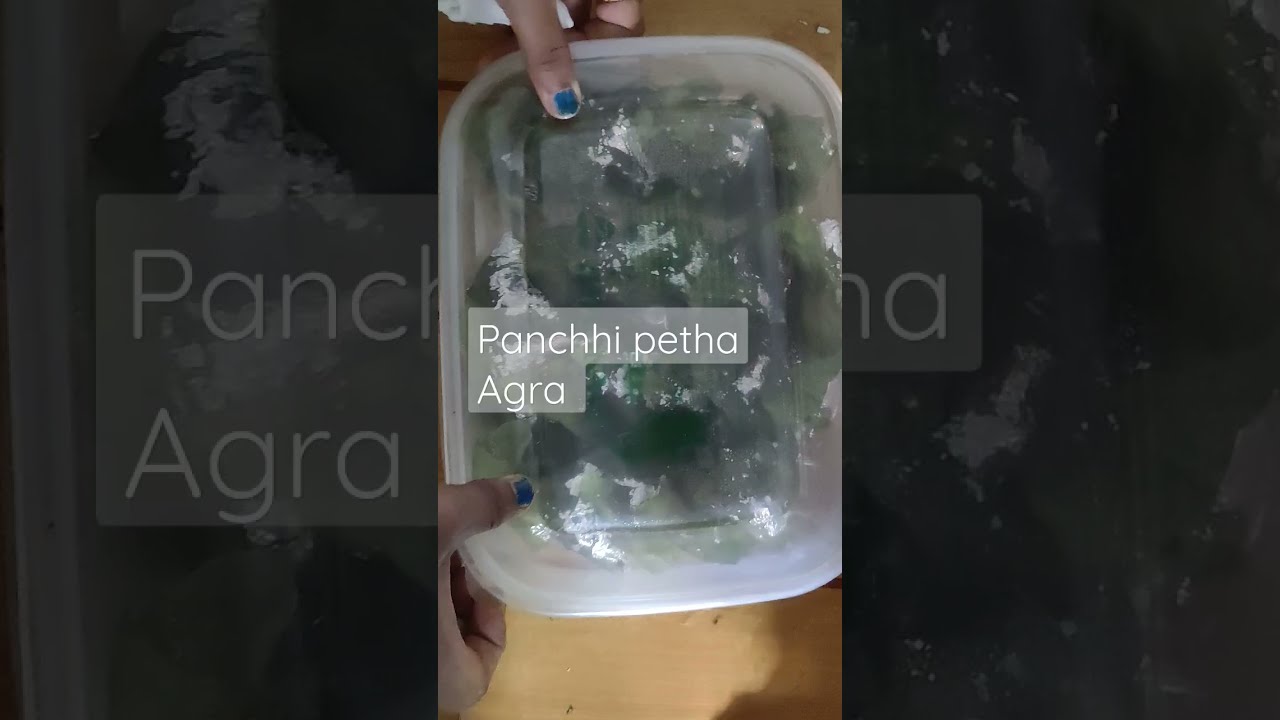The image features a tan background with a central plastic container that nearly fills the frame. The container appears to have various contents and is labeled "Panshi Petha Agra" in text positioned at the top of the image. On the left side of the container, a person with darker skin and blue fingernails is holding the lid, with their fingers visible at the top left and bottom left corners. The container itself shows some black spots, which might be interpreted as soot. The colors present in the image include light brown, tan, white, gray, green, and blue, suggesting a diverse and vibrant palette. The overall style of the image implies that it could be a screenshot from a mobile device.